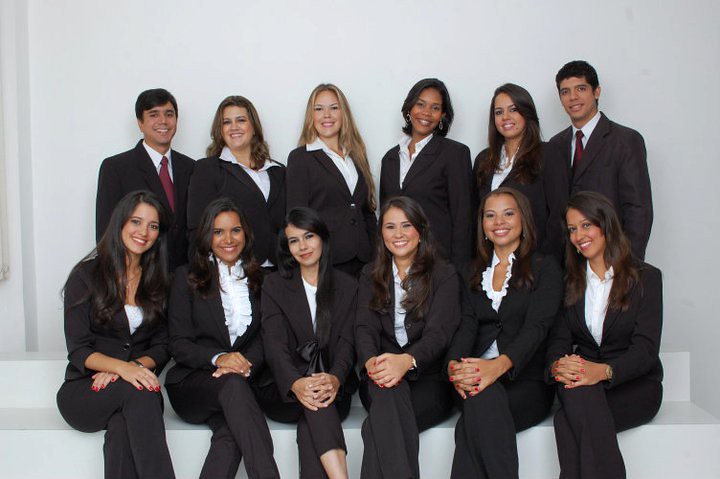The photograph captures a structured group of twelve well-dressed individuals posed in two rows against a pristine white backdrop. The front row features six young women seated on a white bench, each dressed in a black suit paired with a white shirt—some with collars and some with v-necks. The women, characterized by their long dark hair, are smiling and have their hands gracefully clasped in front of them with their legs crossed. In the back row, six individuals are standing: two men positioned at each end wearing black suits with red ties, while the four center figures, all women, mirror the attire and smiles of the seated women. The setting appears to be an indoor professional environment, devoid of any visible text, with the individuals prominently centered in the image, exuding a cohesive and polished appearance.